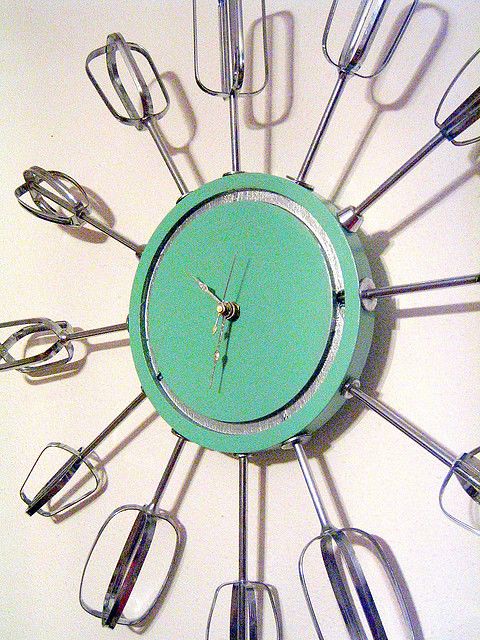This image captures a uniquely designed kitchen clock, creatively crafted from green round objects. The clock face consists of a green circle with elegant silver hands that point to the time. A silver trim frames the central green circle, enhancing its aesthetic appeal. The photo is taken from a side angle, which beautifully highlights the clock's depth and structure, featuring a pronounced lip. Adorning this lip are silver beaters resembling those found in an automatic mixer, subtly indicating the clock's kitchen theme. Multiple shadows on the wall suggest the presence of a light source illuminating the area, adding a dynamic and lively dimension to the image.